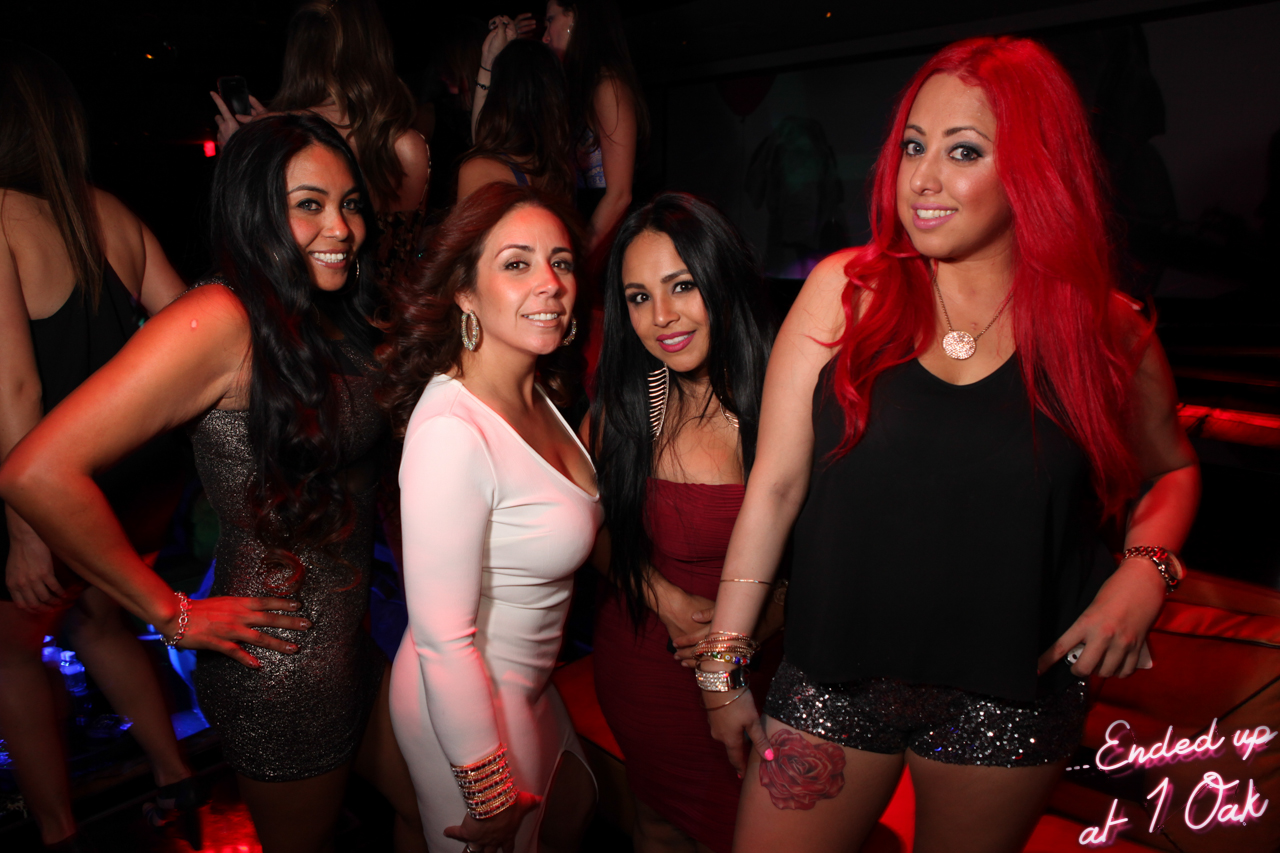In this lively nightclub photograph taken indoors, four young women pose for the camera, each with unique and eye-catching styles. Starting from the right, a woman with vibrant red hair, possibly dyed, flaunts sparkly black shorts paired with a black tank top. Her look is accessorized with a round pendant necklace and assorted bracelets, while her right thigh displays a striking rose tattoo.

To her left stands a woman in a dark, possibly maroon, dress. She has long black hair cascading down and holds her hands neatly in front of her. Next is a woman in a white dress with a plunging neckline and a V-shaped bottom hem that reveals part of her leg. Her look is completed with hoop earrings and gold bracelets adorning her right wrist.

On the far left, a woman in a short, sparkly black dress positions her right hand on her hip. She, too, has long black hair reaching her waist. In the background, the dimly lit setting reveals other club-goers, some with their backs to the camera, enhancing the crowded, festive atmosphere. In the bottom right corner, a neon sign caption reads "ended up at One Oak," hinting at their glamorous location presumably within the Mirage Hotel in Las Vegas. All four women are smiling, exuding a sense of joy and camaraderie as they enjoy their night out.